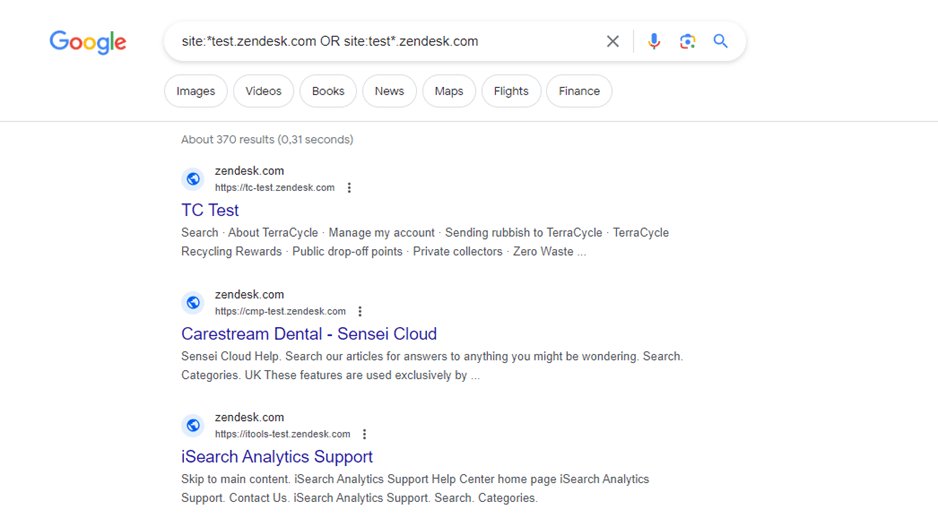This image captures a Google search query demonstrating results for specific Zendesk-related sites. The search input field contains "site:*test.zendesk.org OR site:test*.zendesk.com" in capital letters. The Google search engine has returned approximately 370 results in 0.31 seconds.

The first result highlights "TC Test" and includes references to "TerraCycle." Detailed descriptions under this result mention topics like "Manage accounts," "Sending rubbish to TerraCycle," "TerraCycle recycling rewards," "Public drop-off points," "Private collectors," and "Zero waste."

The second listed result is "Carestream Dental Sensei Cloud," though no further details are provided within the image.

The third and final result is "iSearch Analytics Support." This entry contains various navigational prompts such as "Skip to main content," "iSearch Analytics Support Help Center homepage," "iSearch Analytics Support Contact Us," and "iSearch Analytics Support Search categories."